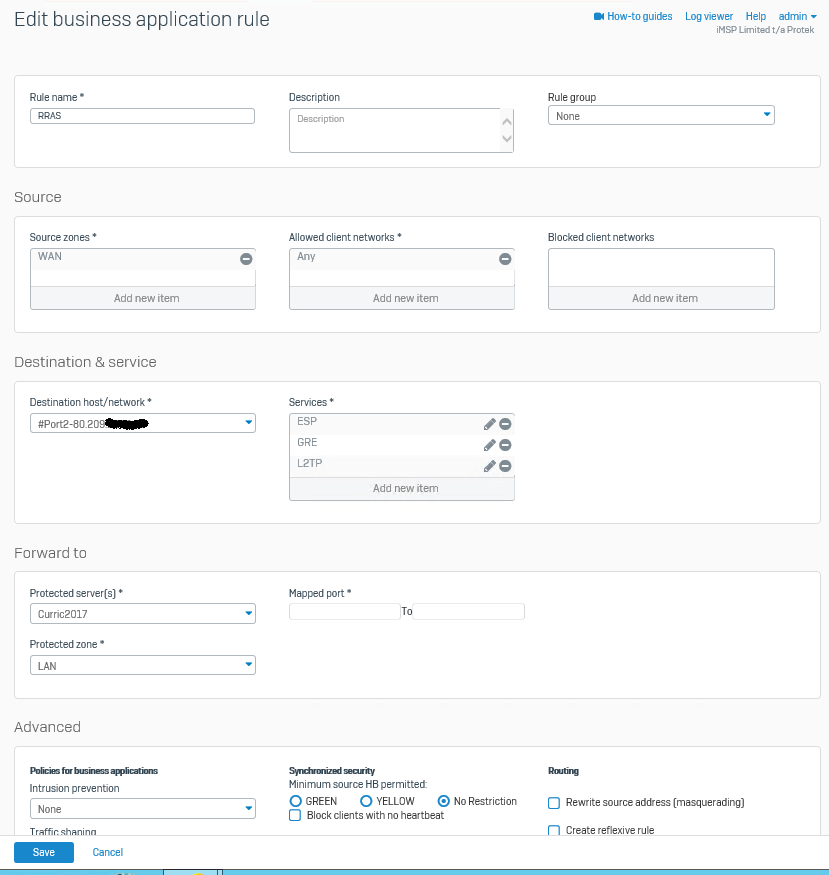This image depicts a detailed screenshot of a computer interface for editing a business application rule. At the top of the page, there is a white rectangular area titled "Edit Business Application Rule," which includes fields for "Rule Name," "Description," and "Rule Group." Within this section are various smaller rectangles designed for inputting information. 

In the blue navigation bar above, clickable links labeled "How to Guides," "Log Viewer," "Help," and "Admin" are visible, with the "Admin" link featuring a dropdown arrow.

Below this, within a section labeled "Source," are three adjacent rectangles named "Source Zones," "Allowed Client Networks," and "Blocked Client Networks." As you scroll further down, there is another rectangle labeled "Destination and Service," containing two additional rectangles. The first is for "Destination Host/Network," and the second, a larger and wider rectangle, is for "Services." Notably, someone has used a black pen to cross out numbers in the "Destination Host/Network" box.

At the bottom of the interface, more input boxes are visible, culminating with a blue "Save" button located at the lower left corner of the page.